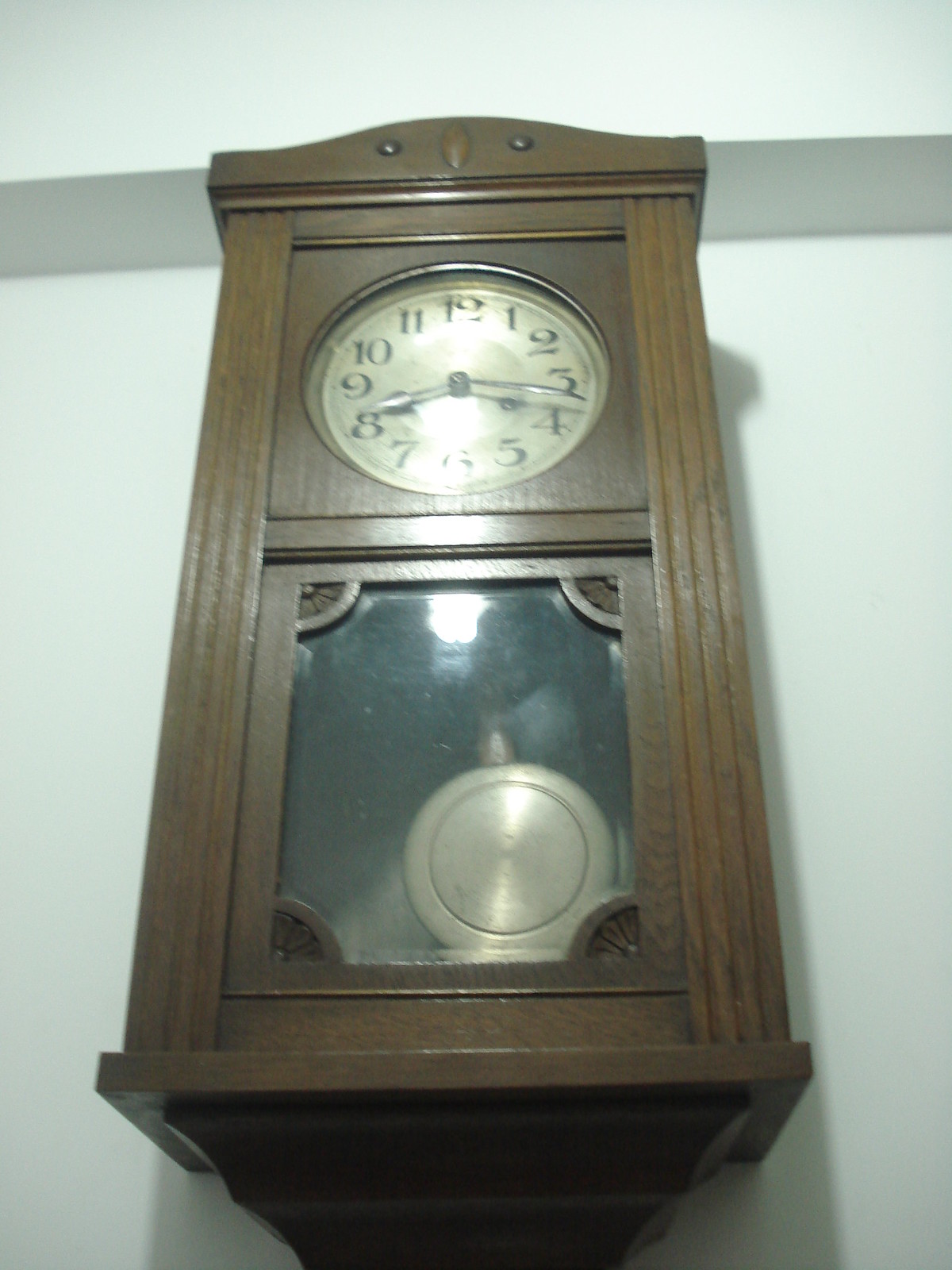This indoor color photograph captures a wall-mounted, rectangular wooden clock with a dark brown, possibly mahogany, frame and a slight upward arch at the top. The clock exudes an antique charm reminiscent of a 1970s style, with its tall structure likely spanning from the tip of a finger to an elbow. The upper half of the clock features a round clock face set in a square panel, displaying black numerals and black hour and minute hands against a silver background, indicating the time as 8:18. The bottom half houses a glass panel, offering a clear view of the large brass pendulum, swung to the right, that swings back and forth and is attached to a rod. The white wall backdrop emphasizes the clock's vintage elegance. No text or print is visible in the image.